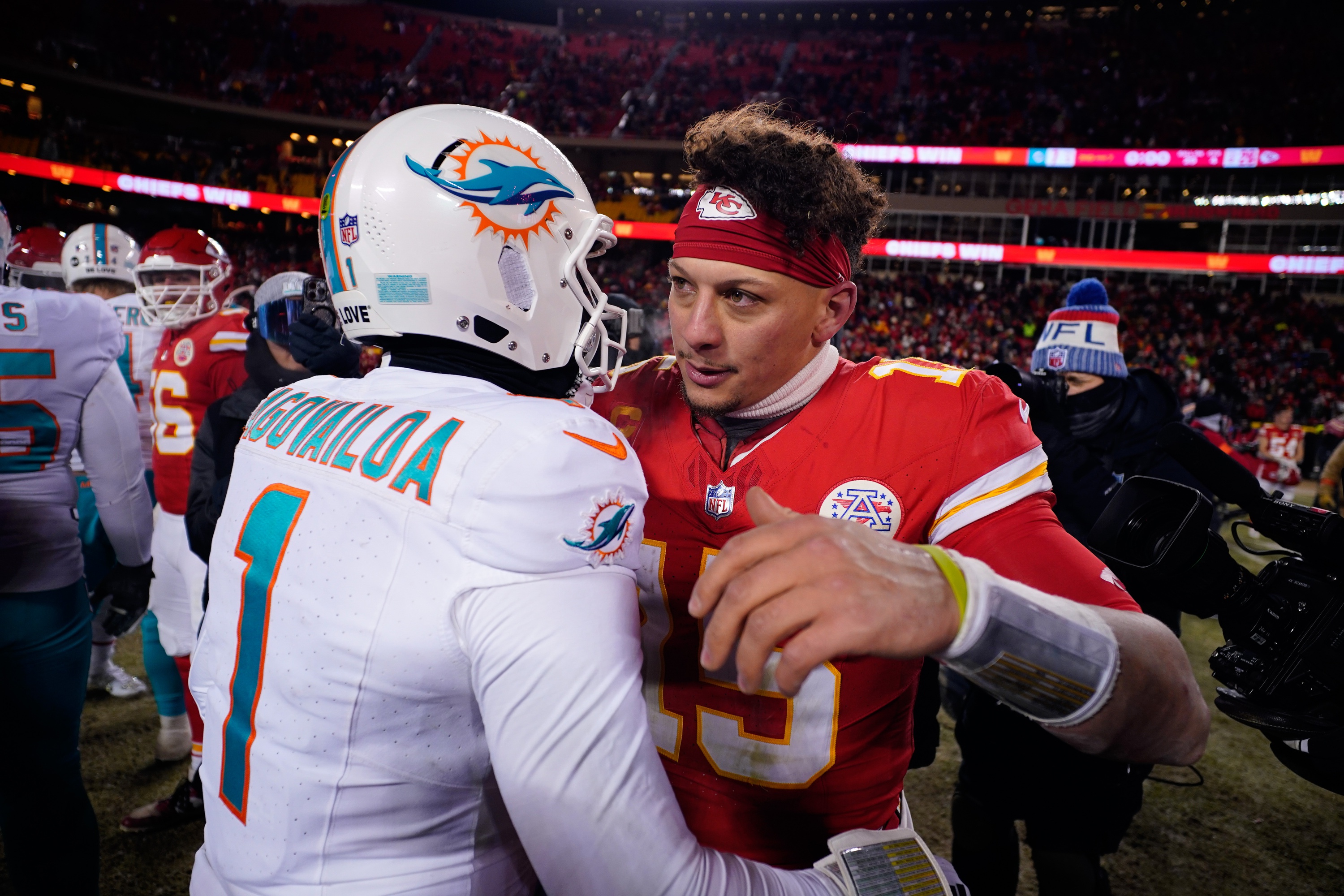In this vivid image from a football game, two players stand prominently in the foreground in a crowded stadium. The player on the left, Tua Tagovailoa, dons a white Miami Dolphins uniform with a blue dolphin emblem on his helmet and a blue number one on his back. He's wearing a white Dolphins cap and a helmet. The player on the right is Patrick Mahomes, dressed in a red Kansas City Chiefs uniform with a red bandana that reads "KC" around his head. Mahomes's arm, slightly dirty, is raised as he begins to embrace Tagovailoa. Surrounding them are additional players from both the Dolphins and the Chiefs. On the right, a person dressed in black pants and a shirt can be seen wearing an NFL cap. In the background, the packed bleachers wrap around the stadium, illuminated by strips of lights at the top.